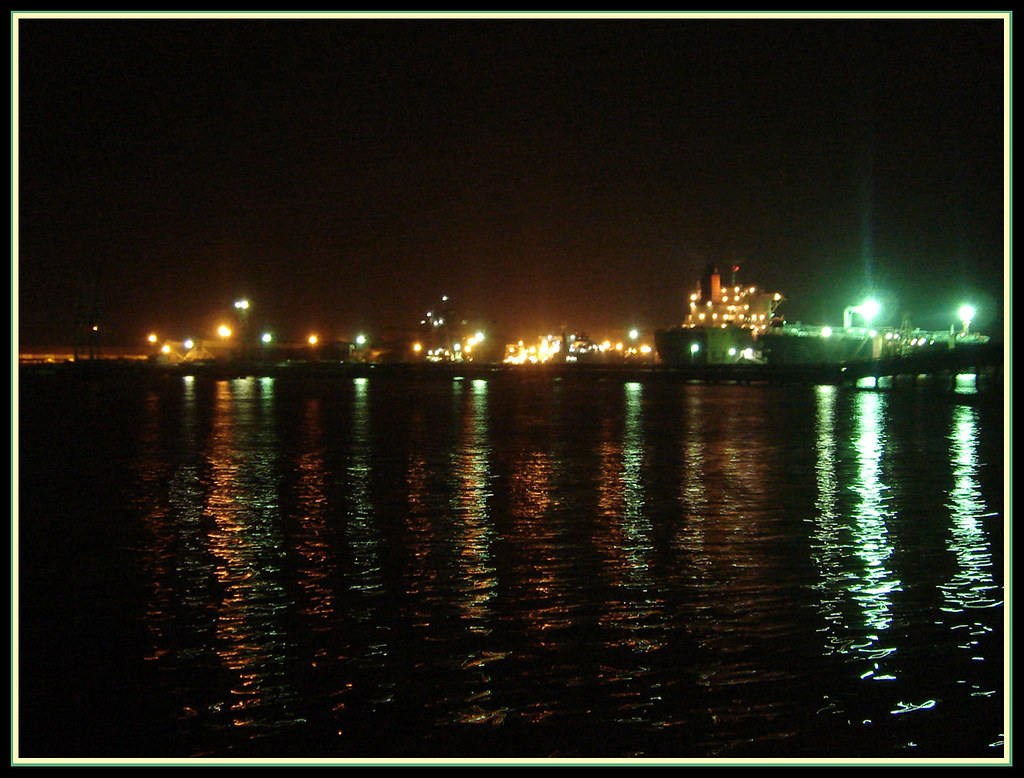The image captures a vibrant nighttime cityscape viewed from across a calm body of water, possibly a lake or harbor. The water in the foreground is smooth, with gentle ripples reflecting the myriad of bright, colorful lights from the city. Among the array of illuminated buildings, a particularly large structure with a striking green spotlight stands prominent on the right. Some shorter, equally radiant buildings fill the center of the scene. The far-right side of the image also reveals a boat adorned with lights, anchored in the harbor. The sky above is a deep black, contrasting dramatically with the glowing landscape below, further enhancing the reflections dancing on the water's surface. Tiny details, like the shimmering lights on the water, add to the image's enchanting nighttime allure.